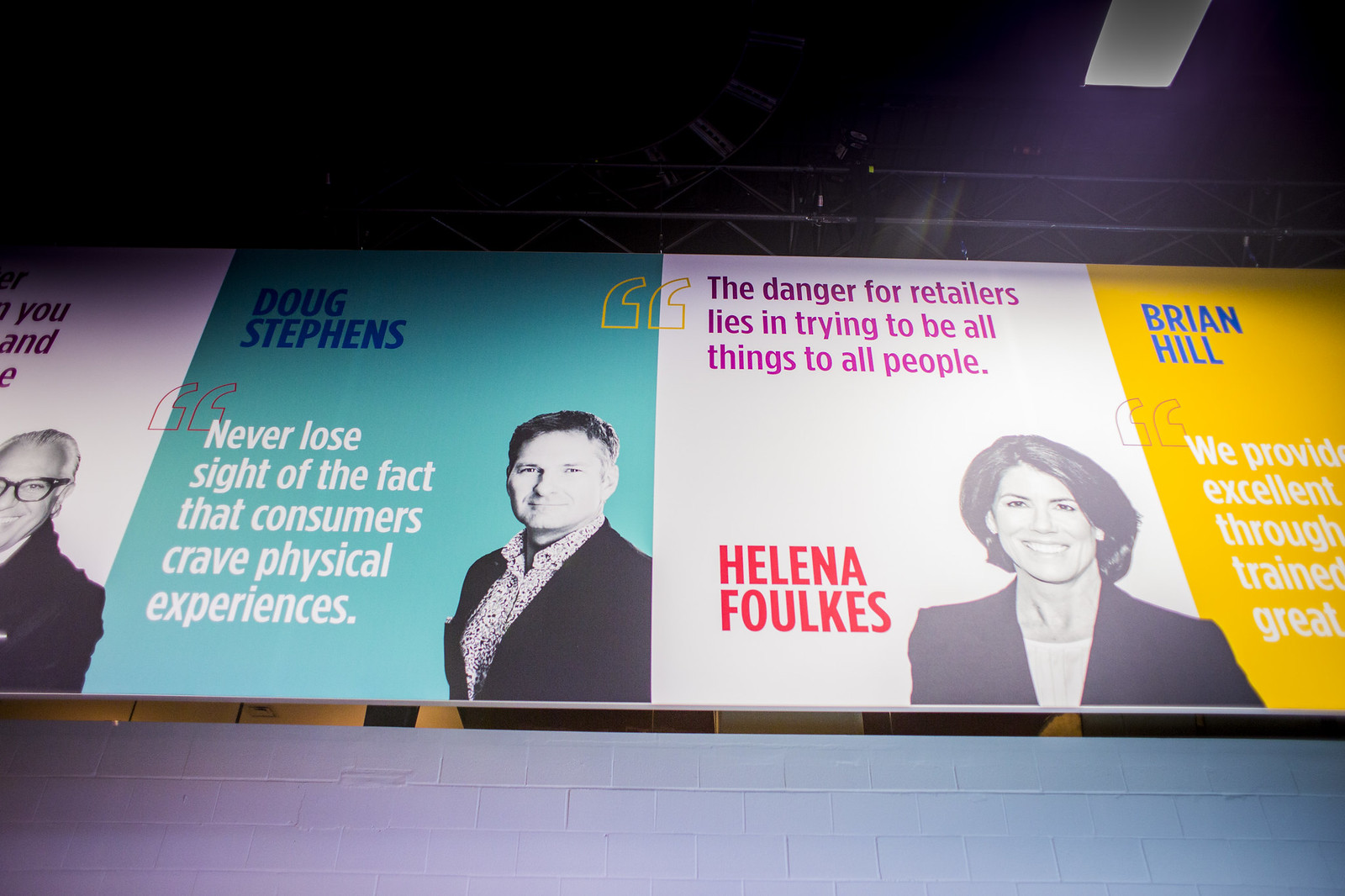The image captures a color photograph in landscape orientation, showcasing a horizontal banner suspended from a dark ceiling. The banner features multiple depictions of people along with quotations attributed to them. Dominating the center of the image are two fully visible sections. 

On the left, the section has an aqua background with Doug Stevens' name in bold blue type at the top left. Adjacent to his black-and-white photo, the white text reads, "Never lose sight of the fact that consumers crave physical experiences." 

To the right of this is another section with a white background. The quotation in pink at the top reads, "The danger for retailers lies in trying to be all things to all people." Below the quotation, there is a black-and-white photo of a woman with short dark hair, identified by the dark red text as Helena Foulkes.

The overall photographic style can be described as representational realism, with additional partially visible sections flanking the two main featured individuals, indicating a broader array of portraits and quotations on the banner.